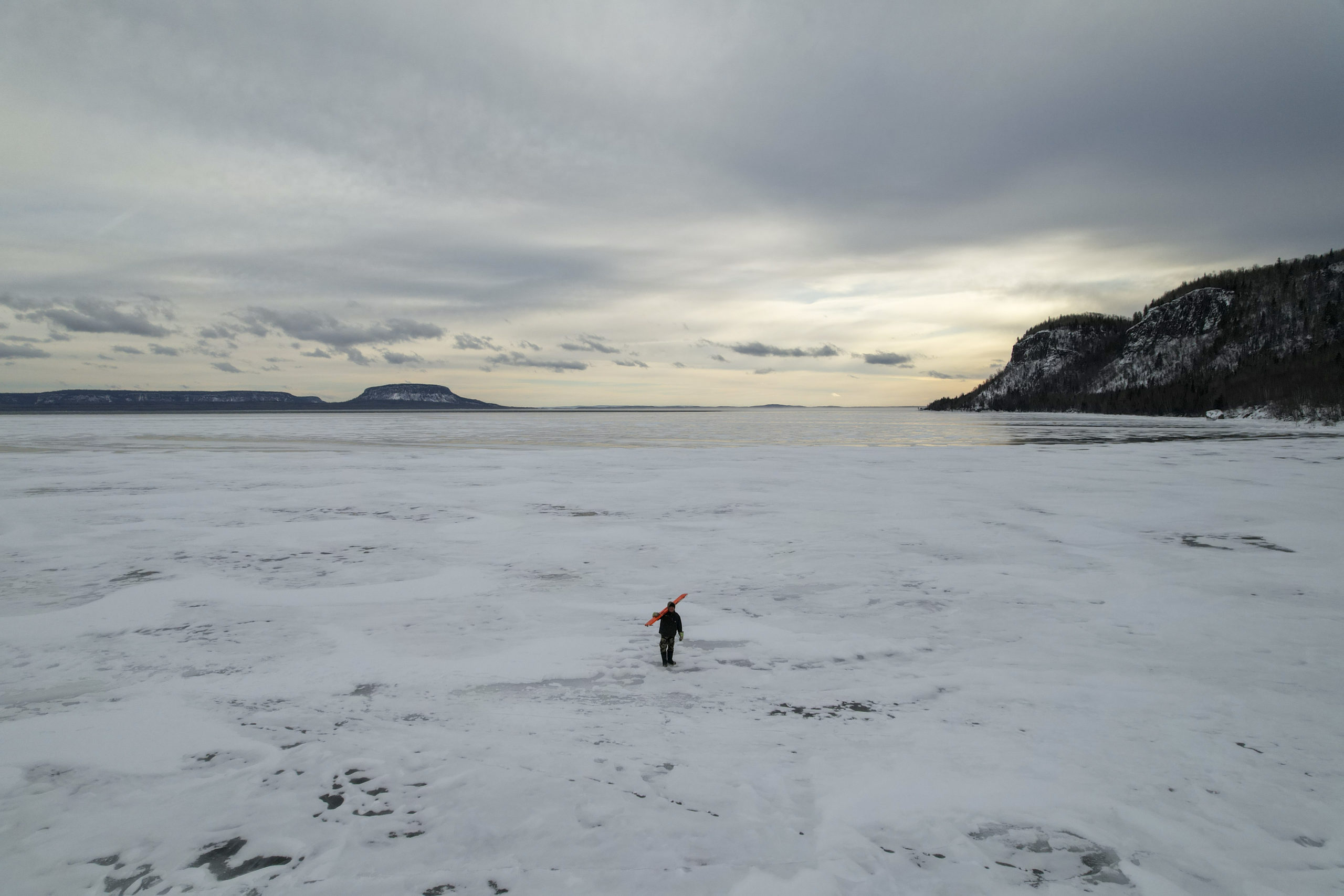The photograph captures a distant man walking across a vast, snow-covered field, possibly in an Arctic environment. He is dressed warmly in a long winter jacket, winter pants, gloves, winter hat, and boots, and he carries a pair of orange skis over his right shoulder. The expansive, white snowy field dominates the lower half of the image, while the man, located in the lower third of the picture and small due to the distance, faces the camera. In the background, a tranquil body of gray water stretches across the middle of the scene, devoid of waves. To the right, dark hills with patches of snow rise from the shore, and similar hills are visible on the left side of the image. The sky above is heavy with gray clouds, reinforcing the wintery, possibly Arctic, atmosphere of the scene.